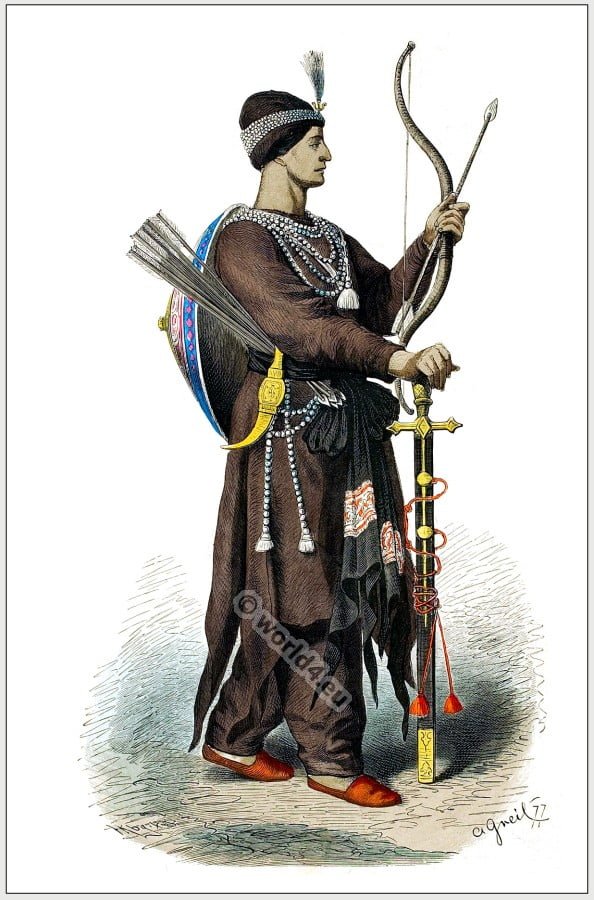The image is a detailed hand-drawn illustration against a white background, showcasing a man of Asian descent. He is dressed in a long, brown cloak and matching turban adorned with pearls and beads. A small feather sticks out from the front of his headdress. Around his neck, he wears several white bead necklaces, and more beads embellish his waist. The man is equipped for battle, holding a brown bow in his left hand and a sheathed sword in his right, which he presses against the ground as if using it as a cane. The sword's sheath is intricately decorated with red rope and gold outlines. On his back, he carries a colorful shield-like item that features a pattern of blue and pink with stripes and diamonds, along with a large hat resembling an Asian field worker’s hat. His footwear consists of bright red shoes.

On the ground below him, a small cream-colored pavement is visible. The backdrop remains plain and white except for shades of grass at his feet and a distinctive signature reading "A-G-N-E-I-L 77" in the bottom right corner. Additional details include a black belt around his waist holding a quiver filled with arrows, and he appears to be ready for either defense or confrontation. The illustration is detailed and colorful, making it an engaging and vivid representation, possibly from a historical or mythical era. This artwork is copyrighted by World4EU.